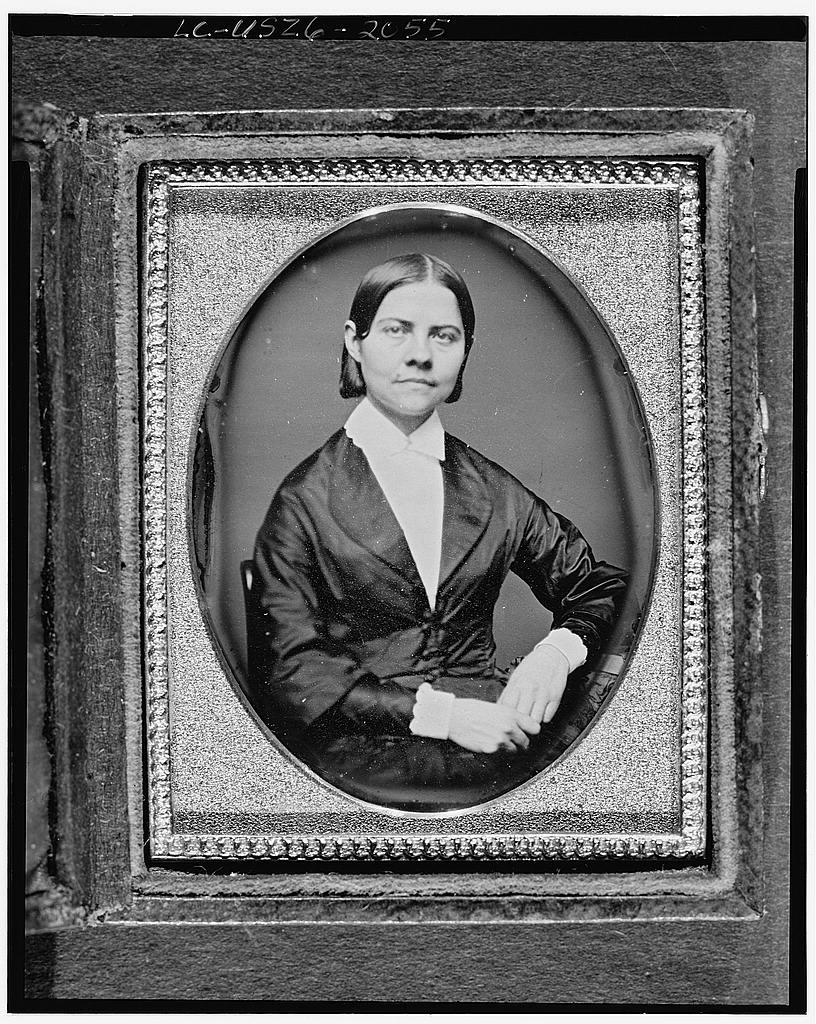This is an intricately detailed black-and-white photograph of a woman, seemingly taken in a bygone era. The central figure, a middle-aged woman, wears a white collared shirt with white frilled cuffs under a black jacket. She has a pleasant expression and her hands are crossed over her waist as she appears to be seated, her right elbow resting on her lap. Her hair is short, black, and parted down the middle, reaching the nape of her neck. The photo itself is enclosed within an oval opening, which is part of an ornately designed, bejeweled-looking case. This silver-patterned frame is encrusted with jeweled rocks, giving it an exquisite and elegant appearance. The case is nested within a secondary larger frame, possibly made of leather or metal, that adds multiple layers to the overall presentation, making it seem as though the image is part of a fold-out book or a treasured keepsake.